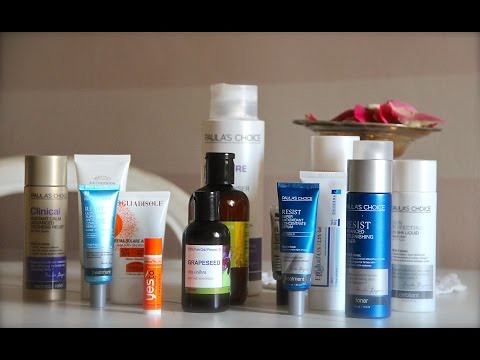On display is a collection of 14 skincare items, primarily from Paula's Choice, set against a brown background with a lighter strap running horizontally through the center. The arrangement showcases a variety of tubes and bottles, each detailed with unique labels and colors.

Starting from the left, the first item is a brown tube with a blue label at the bottom, likely from Paula's Choice's clinical line. Next to it, a shiny light blue tube catches the light, followed by a white tube that features an orange circle and red rectangular shapes with text at the bottom. A small cylindrical tube resembling chapstick stands out with its mostly orange design and the words “Yes To” partially visible on its side.

To the left, there's a dark bottle with a white square label that reads "Grape Seed," and behind it is another dark bottle with a green label. At the back, an item wrapped in plastic bears the Paula's Choice branding. Moving rightward, one finds a Paula's Choice Resist product in a light blue metallic tube adorned with a silver strip.

Further to the right, a white tube with more text and an adjacent Paula's Choice Resist item with a silver cap are visible. Immediately next to this is a white bottle labeled "Paula's Choice," mentioning a liquid product with additional text and a signature.

The visual theme of these items revolves around skin tones, complemented by a decorative bowl in the background filled with red flower petals, enhancing the aesthetic appeal of the display.